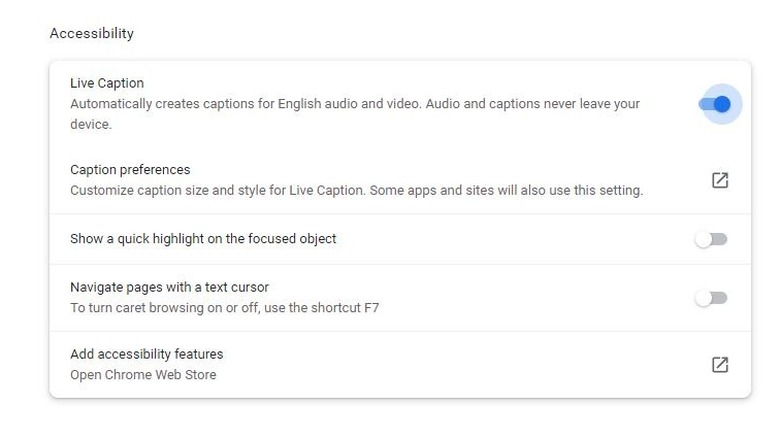The image depicts a user interface focused on accessibility features against a gray background. At the top, the title "Accessibility" is prominently displayed. 

Within the white box:
- In the top left corner, the feature "Live Caption" is introduced with a description underneath stating, "Automatically creates captions for English audio and video. Audio and captions never leave your device." To the right of this text is a toggle switch, which is illuminated in blue, indicating that Live Caption is currently enabled.

- Following a line break, the section "Caption Preferences" appears. Below it, the text reads, "Customize Caption Size and Style for Live Caption. Some apps and sites will also use this setting." Adjacent to this description is a clickable box with a line running through it, indicating a setting option.

- A light gray horizontal line separates this from the next section: "Show a quick highlight on the focus object," accompanied by a toggle switch to the left, turned off and colored gray.

- Another light gray horizontal line follows, leading to the final option: "Navigate pages with the text cursor. To turn caret browsing on or off, use the shortcut F7." This setting also features a toggle switch on the left, currently turned off.